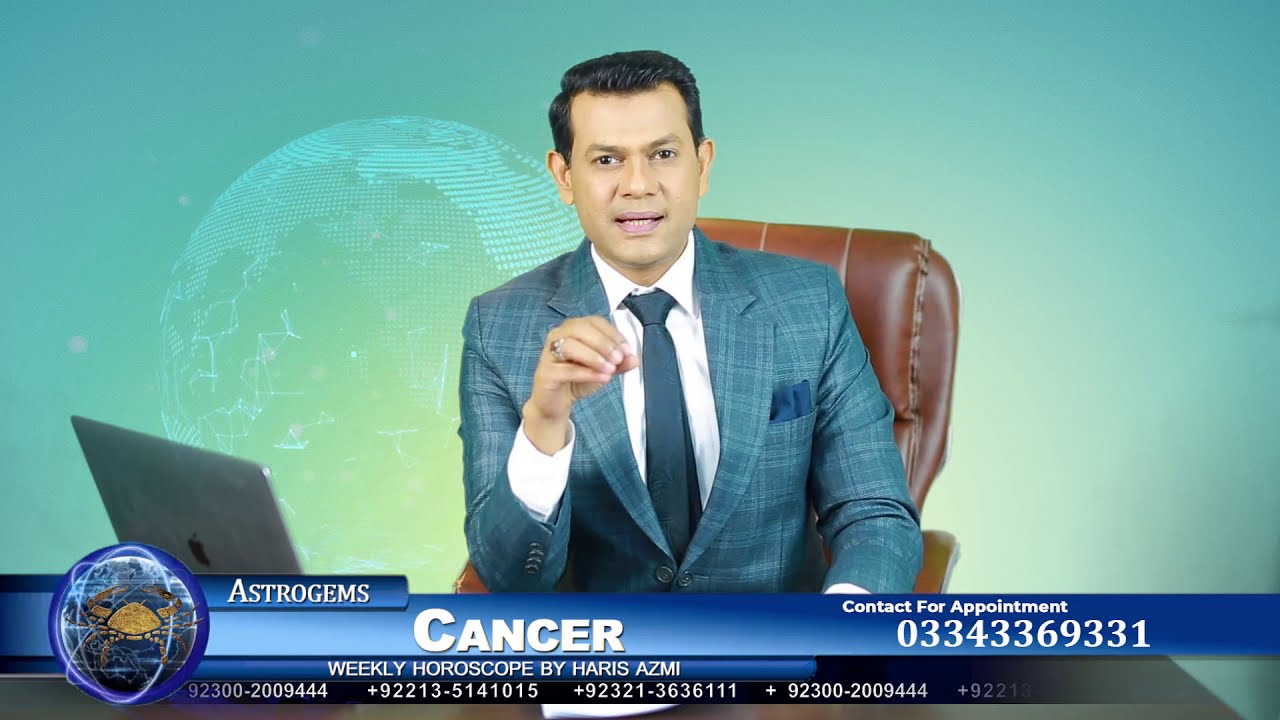This horizontal rectangular image seems to be an advertisement featuring a man of possibly Mexican descent seated at a brown leather desk chair behind a wooden desk. The background is green with a circular outline resembling a globe, consisting of white computerized dots. The man, who has short black hair, is looking directly at the camera with his mouth slightly open as if speaking. He is dressed in a plaid blue suit jacket with a navy blue tie and a white button-down collared shirt, complete with a blue pocket square. His right hand is raised in front of him, and he is wearing a ring on that hand. To his right sits an open Apple laptop.

At the bottom of the image, a horizontal blue bar with white text runs from left to right. The prominent text states "CANCER" in all caps, with "Contact for appointment" below it, followed by the contact number "0334-336-9331." Further text in smaller white caps reads "WEEKLY HOROSCOPE BY Harris AJRIS and AZMI." The scene suggests that the man is presenting astrological content.